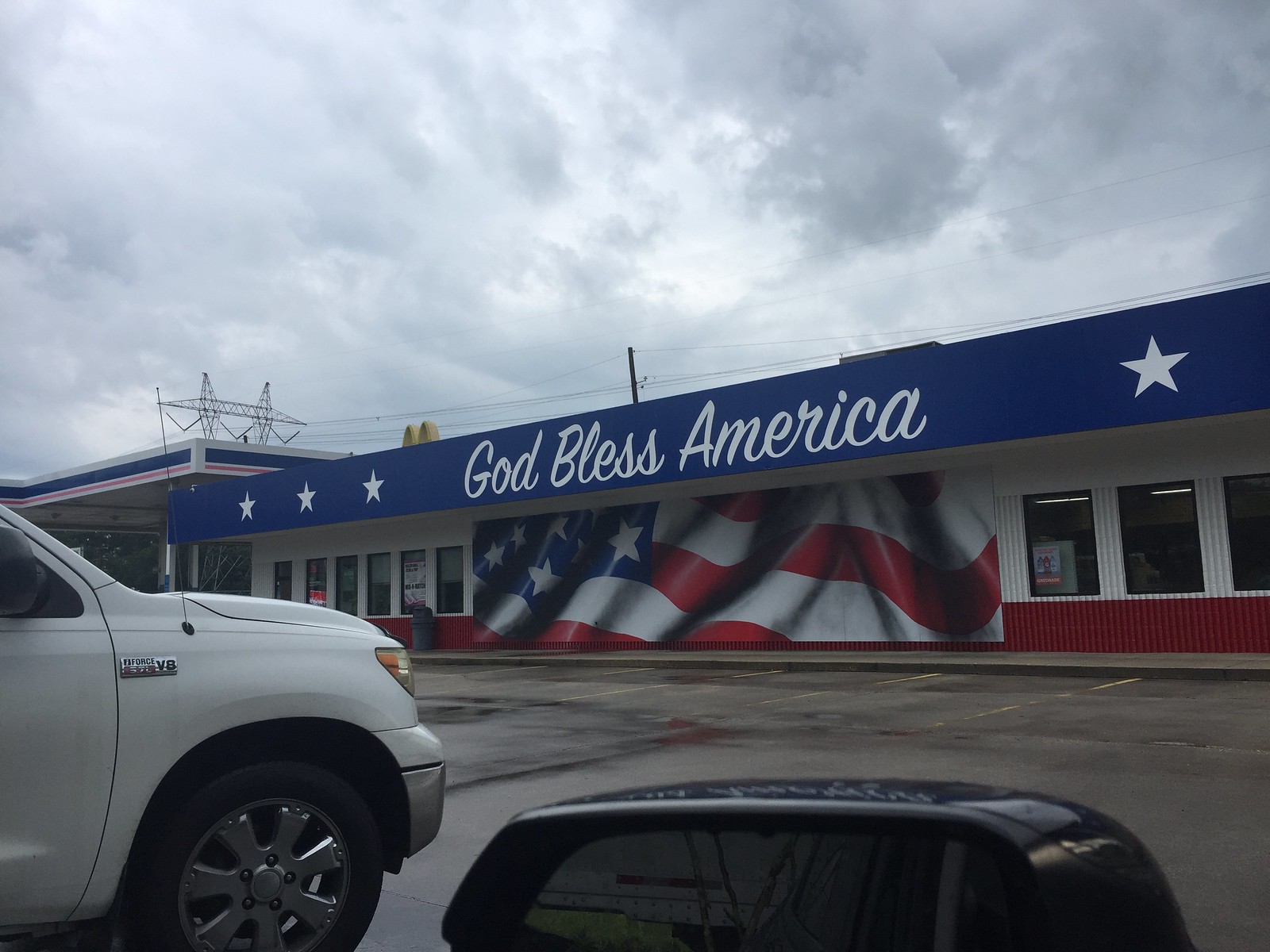The image depicts the exterior of an elongated rectangular building that could either be a restaurant or a retail store. The structure appears to be constructed from either metal or painted concrete and features a flat roof. Prominently displayed on the front is a large sign that reads "God Bless America" in blue with white font, accompanied by three white stars next to "God" and one star next to "America." Just below the sign, a vibrant mural of a billowing American flag adorns the facade. Flanking the mural on either side are windows, and further down the building, partially obscured by a parked car, is a door. Due to the obstructed view, the exact nature of the establishment remains unclear.